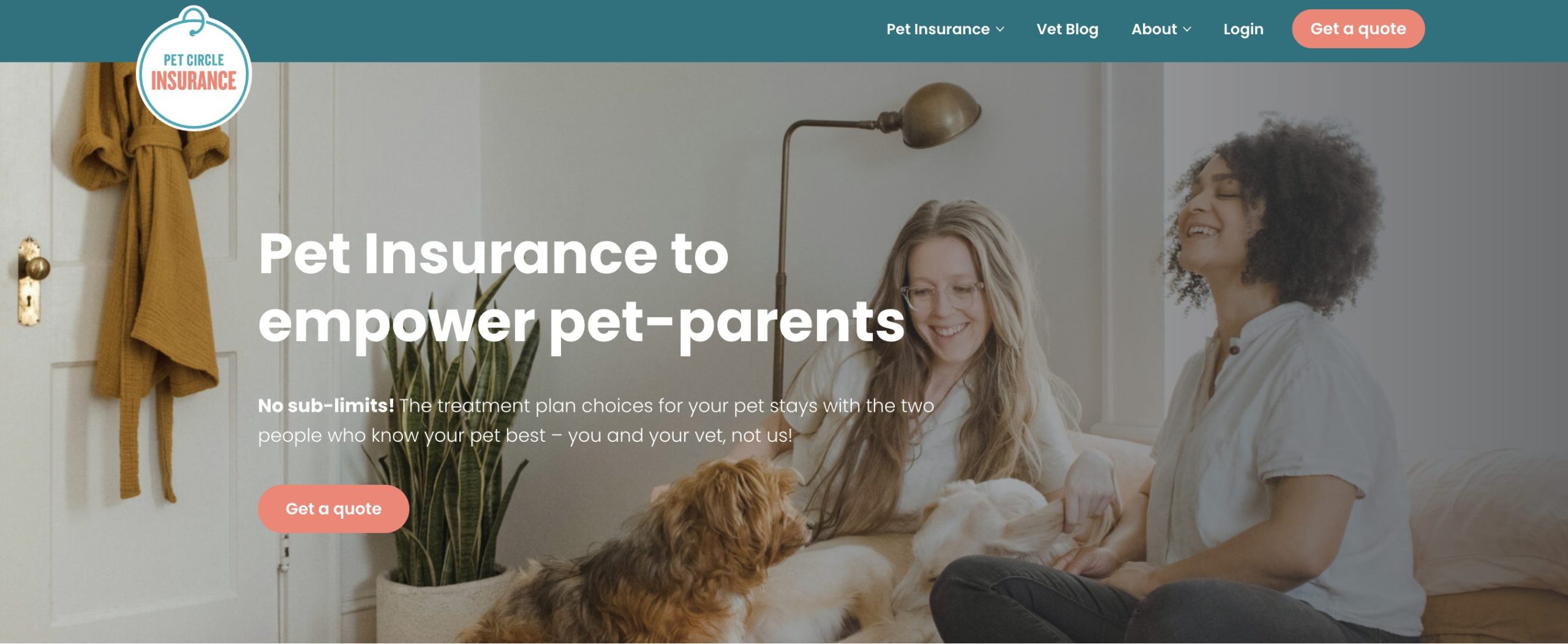The image depicts a splash screen for a website called Pet Circle Insurance. In the top left corner, there is a small circle containing the text "Pet Circle Insurance," with "Insurance" written in orange and "Pet Circle" in a bluish shade. This circle hangs from a blue banner that runs across the top of the screen. On the right side of the blue banner, there are several navigation options: a pull-down menu for pet insurance, a vet blog link, a pull-down menu for information about the site, a login link, and an orange "Get a Quote" button on the far right.

The main splash screen features a heartwarming image of two girls sitting on a sofa with a dog in front of them. To the left of this image, in large white font, the text reads: "Pet insurance to empower pet parents." It further mentions, "No sublimits. The treatment plan choices for your pet stay with the two people who know your pet best, you and your vet, not us."

Beneath this text, there is another "Get a Quote" button in orange, located on the left side of the screen, near where the dog is positioned in the picture. This provides a clear and inviting call to action for users interested in obtaining a quote for pet insurance.